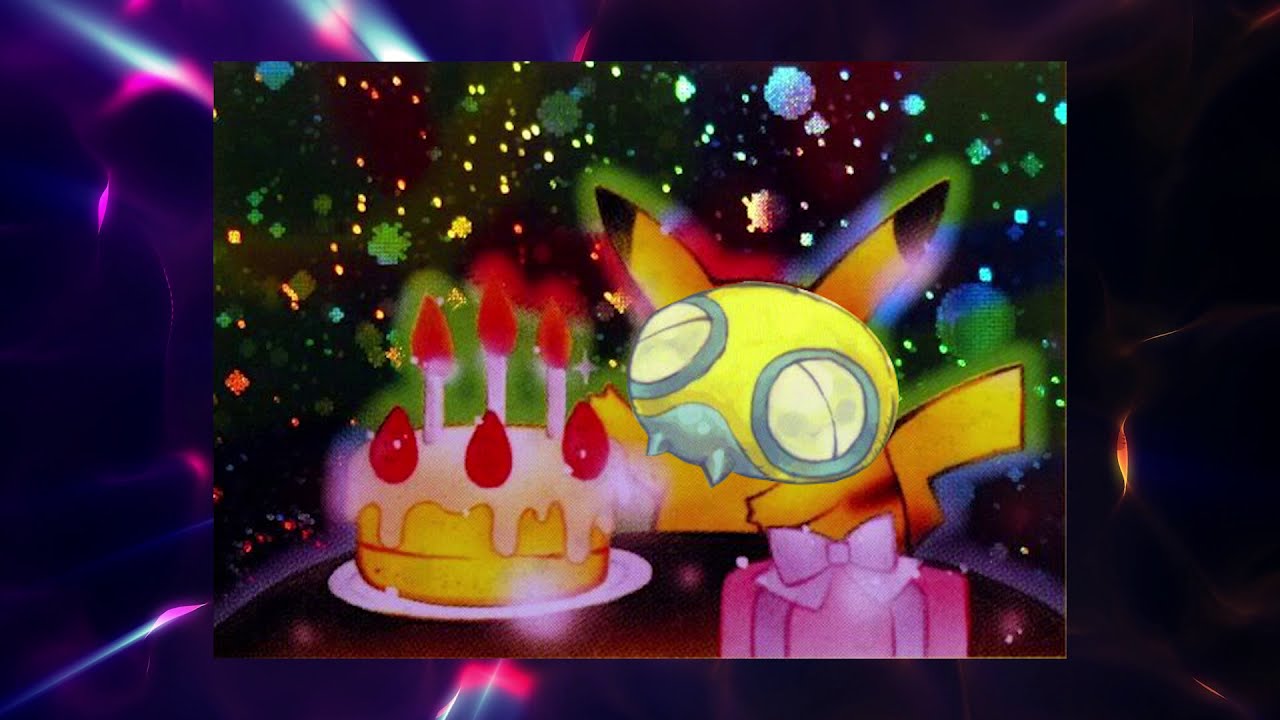This is a horizontally wide digital artwork with a vibrant, neon-infused background encompassing deep dark bluish-purple shades accented by bright pink and neon blue lights flashing in various areas. Centrally placed within this larger image is a smaller rectangular piece depicting a space-like atmosphere characterized by dark reds, yellows, greens, and blues. Within this space-themed backdrop, bright neon and white star-like objects and snowflakes add an ethereal touch. 

At the heart of the image, a round table is the focal point, adorned with a neon-yellow cake with three to five bright red candles illuminating it. Adjacent to the cake is a digital drawing of Pikachu, the well-known Pokémon character. Pikachu's ears, tipped with black, are perked up, and it seems to be wearing an unusual mask, possibly resembling another Pokémon's head, Dunsparce. Pikachu is positioned to the right of the cake, with one hand lifted while the other rests on its chest. A pink present with a bow is near the cake, adding to the celebratory atmosphere. The entire scene is rendered in a digital fan art style, featuring a complex and colorful background with gradients of green, blue, red, and other hues, emphasizing the fantastical and festive setting.